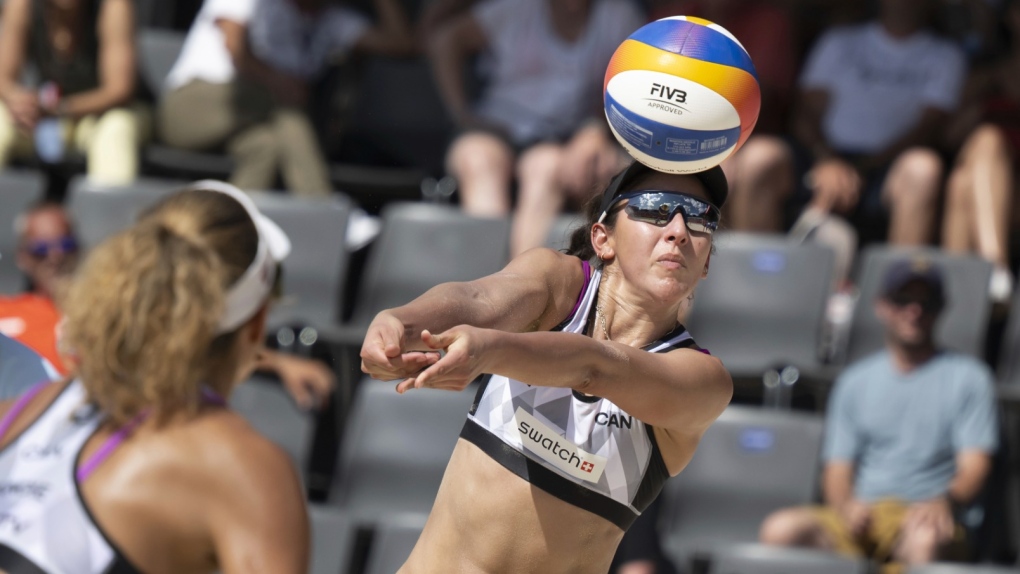This close-up outdoor color photograph captures an intense moment in a women's volleyball match on a bright, sunny day. Front and center is a young white woman, likely in her early 20s, poised to hit a volleyball coming toward her at forehead level. She is wearing reflective sunglasses, a white sports bra emblazoned with the "SWATCH" logo and the Swedish flag on the side, and her dark hair is pulled back. Her arms are outstretched, with her hands positioned to serve or strike the ball, which features white, blue, and orangish-yellow stripes with the words "5 approved" on it. To the left of the frame, another white female player with a brunette ponytail is pictured from the back, wearing a white visor and a sports bra top with purple strings. The background displays a blurred audience seated in the stadium, hinting at the lively atmosphere of the event.